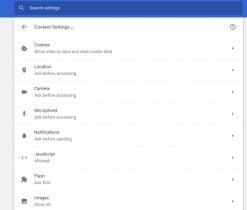This image depicts a low-resolution settings screen with a compact design. At the top, a navy blue bar spans the width of the screen, featuring a magnifying glass icon and the text "Search settings" presumably within a search box. The content below is set against a white background bordered by a faint gray on either side. Despite the small and blurry font, it appears to list various settings categories such as "General Settings" or "Content Settings."

Under this heading, a series of specific settings is listed:
1. **Cookies** - Accompanied by a cookie icon.
2. **Location** - Marked with a GPS logo.
3. **Camera** - Denoted by a camera icon.
4. **Microphone** - Represented with a microphone icon.
5. **Notifications** - Illustrated by a bell icon.
6. **JavaScript**
7. **Plugin** - Highlighted with a puzzle piece icon.
8. **Images** - Identified with a square block icon featuring a small mountain.

Each setting has an arrow icon on the right, either pointing downwards or sideways, indicating expandable options for additional details or configurations.